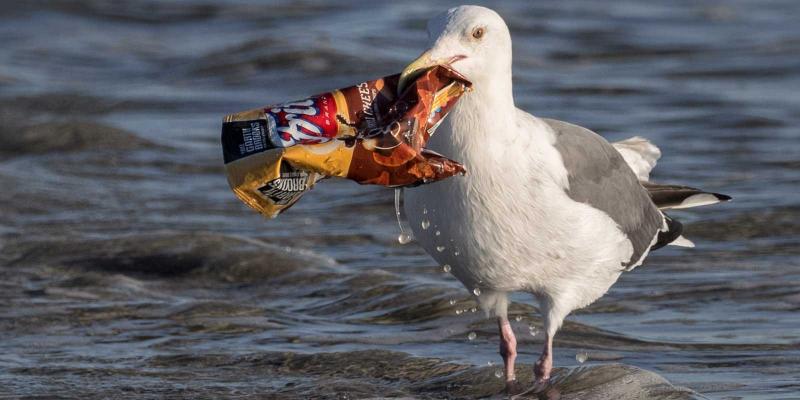This photograph captures a seagull in shallow seawater near the shore, as the water depth only reaches up to the bird's ankles. The seagull, predominantly white with a brown-tan beak, gray wings and tail feathers, and black-tipped tail feathers, stands against a backdrop of bluish-dark gray waves. Its pink legs are visible in the shallow water. The seagull is holding a crumpled, dripping bag of Fritos corn chips in its beak. The Fritos bag, which features a dark yellow-brown bottom and a red label with white lettering, hints at a cheese flavor and includes a Garth Brooks promotion, suggesting the image was taken in America. The bird is positioned facing the left side of the image, and it carries the open, slightly crushed bag in its beak.